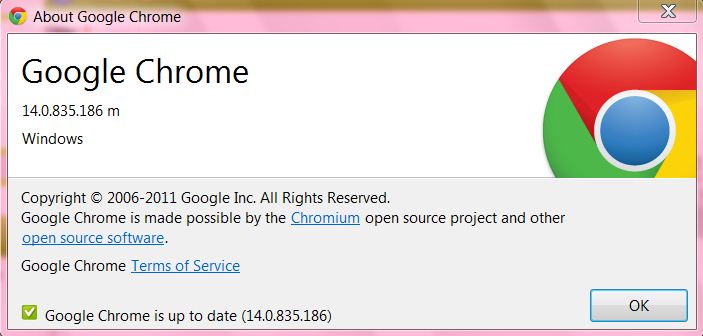This image is a screenshot from a website detailing information about the Google Chrome browser. In the upper left-hand corner, the Google Chrome logo is prominently displayed. The logo consists of a circular design with red on the top, green on the left, and yellow on the right, encircling a blue sphere at the center. Adjacent to the logo, the text "About Google Chrome" is written in black, situated within a pinkish-colored bar.

On the right-hand side of this bar, there is a gray-outlined box with a white 'X' inside, which indicates an option to close the page. Beneath the pink bar lies a white box. At the upper left-hand corner of this white box, "Google Chrome" is written in bold black text. Directly below, it states the version number "14.0.835.186" followed by the letter "M." Further down, the text "Windows" appears in black.

To the right of this text is a larger version of the Google Chrome logo. Below this area, a grayish-colored box contains a copyright notice: "Copyright © 2006-2011 Google Inc. All Rights Reserved," rendered in black text. The statement "Google Chrome is made possible by the Chromium open-source project and other open-source software" follows, with "Chromium" and "other open-source software" highlighted in blue, indicating clickable links.

Continuing down, the text "Google Chrome" is again visible in black, followed by the blue-colored link "Terms of Service." Below this, a green box featuring a white check mark states "Google Chrome is up to date (14.0.835.186)" in black text. To the right, a gray box marked with "OK" provides an option to close the page.